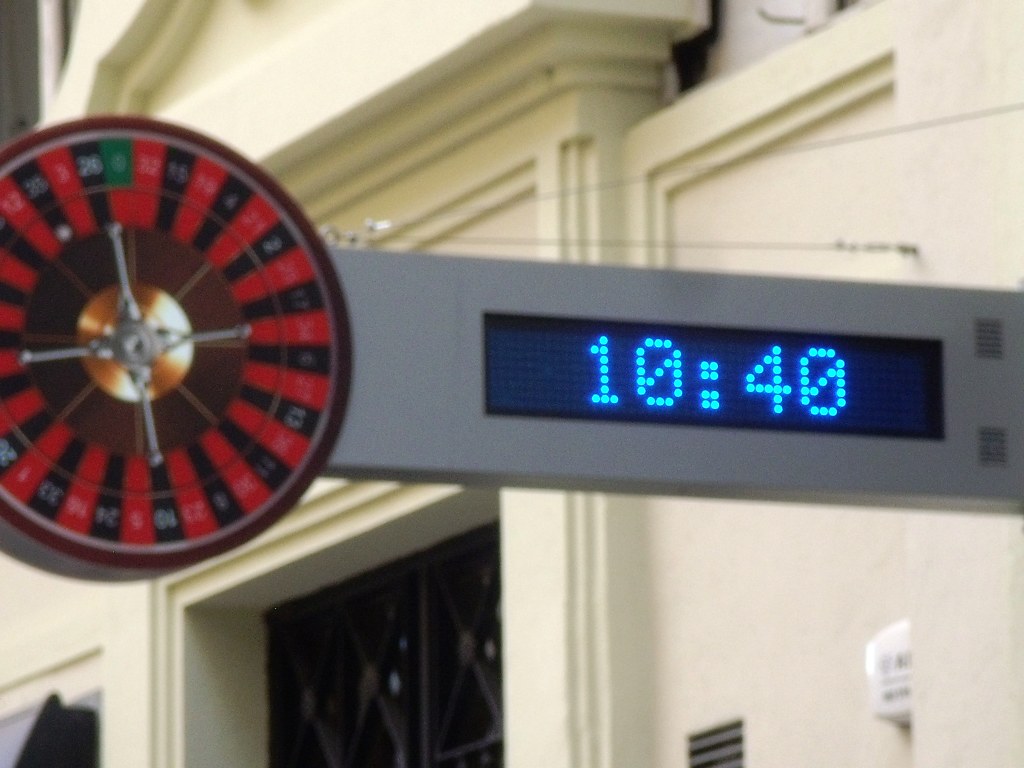The image features a modern digital clock with a blue LED display showing the time as 10:40. This clock is mounted on a grey metal extension that juts out from a plain white wall. At the end of this extension is a vivid, detailed color image of a roulette wheel. The roulette wheel showcases the classic black and red numbered segments, a gold mechanism at its center, and a small white ball, although the numbers on the wheel are too faded to decipher. The background primarily consists of the white wall, with a hint of a black doorway visible, suggesting the setting might be inside a casino.